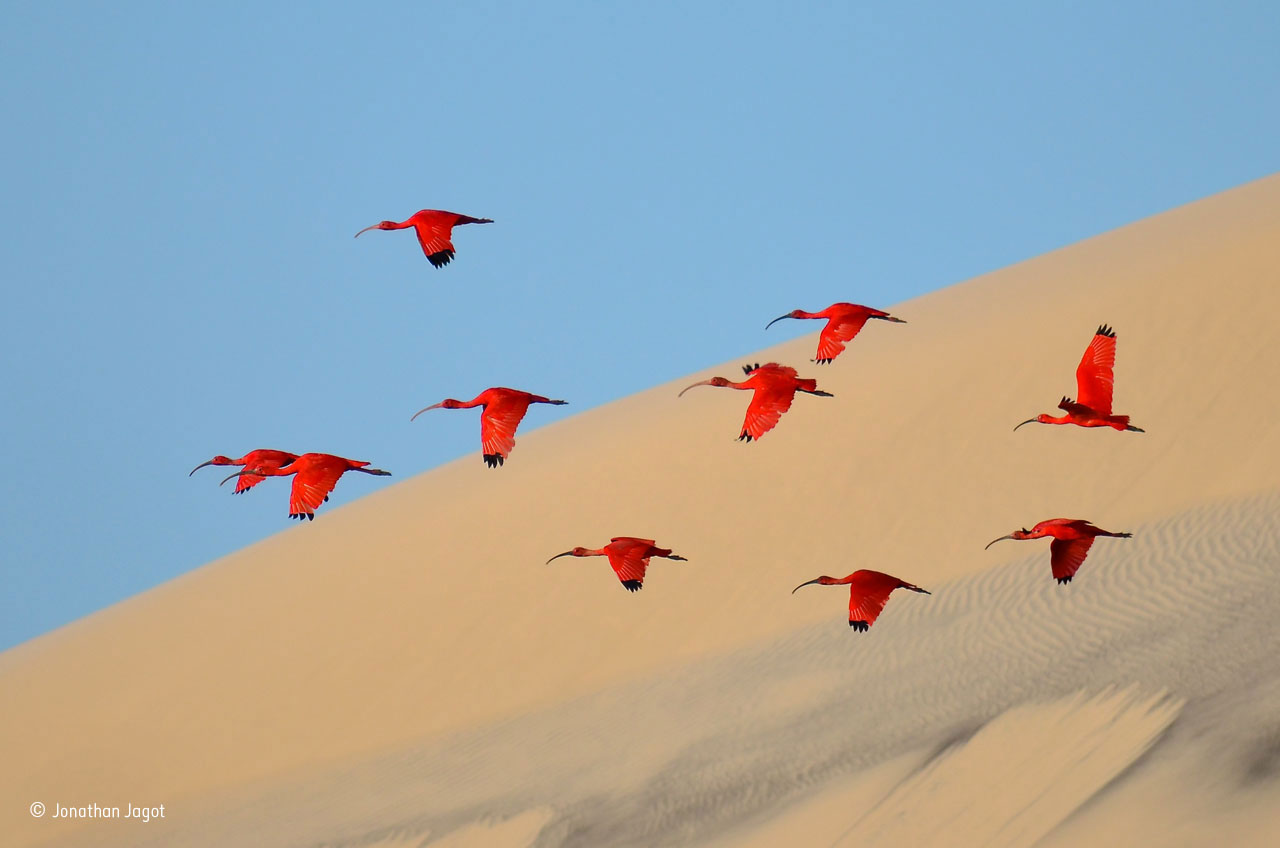In this detailed photograph by Jonathan Jagot, a captivating desert scene is depicted, featuring a stunning contrast between a clear blue sky and vast, rippled sand dunes. In the bottom left corner, the image is marked with Jagot's copyright. The primary focus of the photograph is a synchronized flock of ten vibrant red ibises, identifiable by their long, downward-curving beaks that match the hue of their feathers. The birds' elegant wings are spread wide, revealing striking black-tipped feathers. They soar gracefully from right to left across the photograph, their vibrant colors standing out against the sunlit sand dunes. The serene and bright environment, coupled with the strategic composition of the ibises in flight, creates a visually arresting and tranquil scene, leaving one to ponder the destination of these majestic desert dwellers.